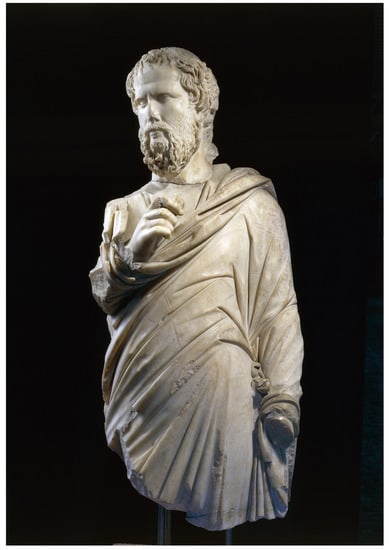The image features a finely detailed Greek statue of a robed man set against a solid black background, emphasizing the sculpture. The statue is intricately crafted from white marble and showcases masterful detailing in the flowing creases of the man's robe. The man's right arm is bent upwards, clutching what appears to be a rock, with the robe wrapped in such a way that it resembles a sling. His left arm hangs by his side, though the hand is conspicuously missing, suggesting it may have been broken off. The statue's head is oriented slightly to the left, revealing a face adorned with curly hair and a luxuriant, curly beard that extends down from his mustache. The figure exudes a contemplative aura, possibly representing a philosopher deep in thought. The lower portion of the statue is cropped out, supported on sticks, and lacks visible legs, leaving its base and original context a mystery.